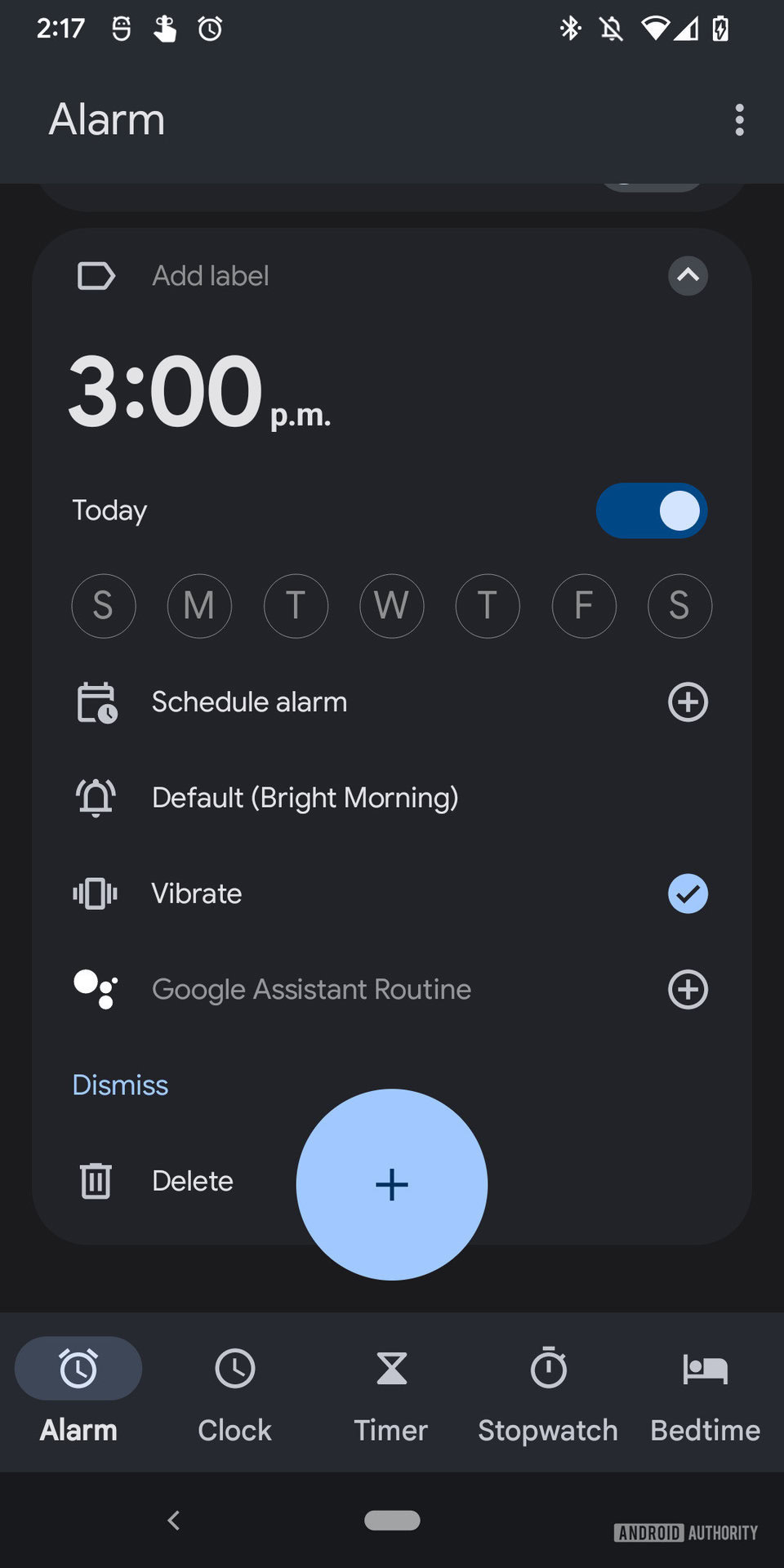This is a detailed screenshot from a mobile phone in dark mode, featuring a charcoal black background. In the upper left corner, the time is displayed as "2:17" in white font. Adjacent to the time are three icons: a finger pressing a button, an "S" icon, and an alarm clock icon. In the top right corner, there is a Bluetooth icon, a bell icon with a slash through it indicating notifications are silenced, a Wi-Fi icon showing four out of five bars of signal strength, a mobile signal icon with three out of four bars, and a battery icon indicating the device is charging.

Below this status bar, there is a gray rectangle with the word "Alarm" in white font. Positioned below that is a large gray square that reads "Add Label" in white font. Centered prominently in large white font is the time "3:00 PM," with the word "Today" displayed just below it. To the right, a toggle switch is visibly set to the 'on' position. Below this setup, there are circles representing the days of the week labeled "S, M, T, W, T, F, S." Finally, at the bottom, "Schedule Alarm" is written in white font.